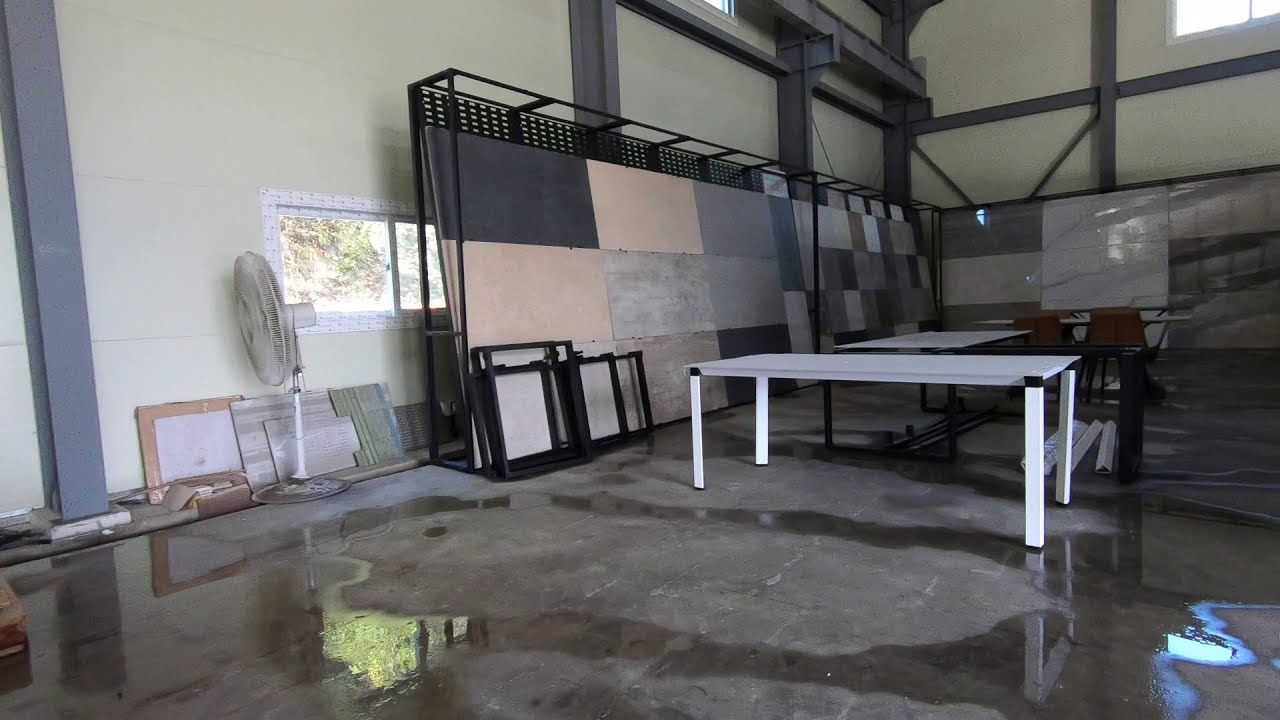This image depicts a large showcase room, possibly in a basement, with light tannish walls and white supports. The floor, covered with noticeable water, suggests a recent leakage or flooding. The central area of the room features several rectangular white tables with four legs, around which few brown chairs are scattered. Towards the left side, there is a prominent white oscillating fan, which seems to be disconnected and leaning against the wall. Adjacent to the fan is a rectangular window with a white frame, through which one can see green leaves and trees basking in sunlight. Additionally, nearby, there are various tiles and rectangular pieces of different colors and textures, including wood and faux marble, possibly used for showcasing flooring or wall designs. The room also includes multiple gray supports extending from the floor to the ceiling.